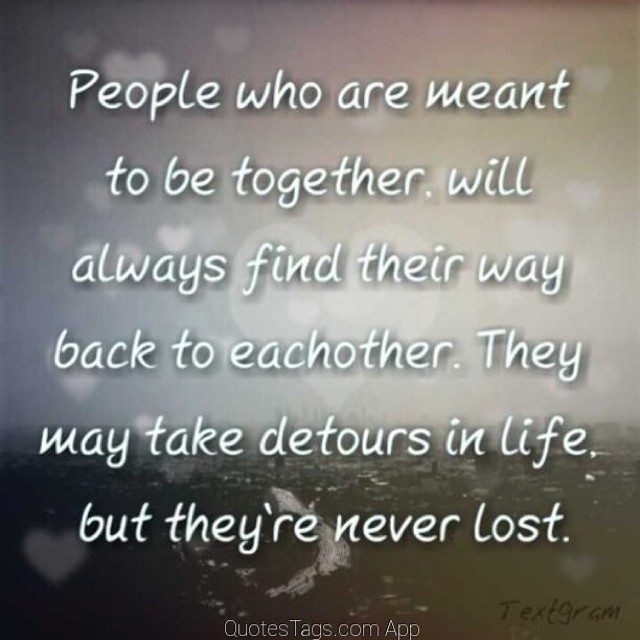This is a perfectly square infographic by QuoteTags.com app, featuring a poignant inspirational quote. The image's background is a grayscale, blurred cityscape with a darker hue at the bottom and a lighter, gray sky occupying the top sixty percent. There are splashes of color faintly visible, including hints of pink, yellow, and blue, interspersed across the background.

Overlaying this backdrop are transparent white hearts, with one large heart centrally placed and numerous smaller hearts adorning the sides, particularly concentrated on the left side. These hearts add a subtle, ethereal element to the image.

Dominating the visual, white sentence-case text, accented by a faint gray drop shadow, reads: "People who are meant to be together will always find their way back to each other. They may take detours in life, but they're never lost." This quote stretches from the top to the bottom of the image, seamlessly blending with the hearts and skyline.

At the bottom center, in small white text, is the acknowledgment "QuoteTags.com app," with the word "Textgram" faintly present in black text to its right. This detailed combination of text, colors, and overlays crafts a visually appealing and emotionally resonant message about enduring connections.